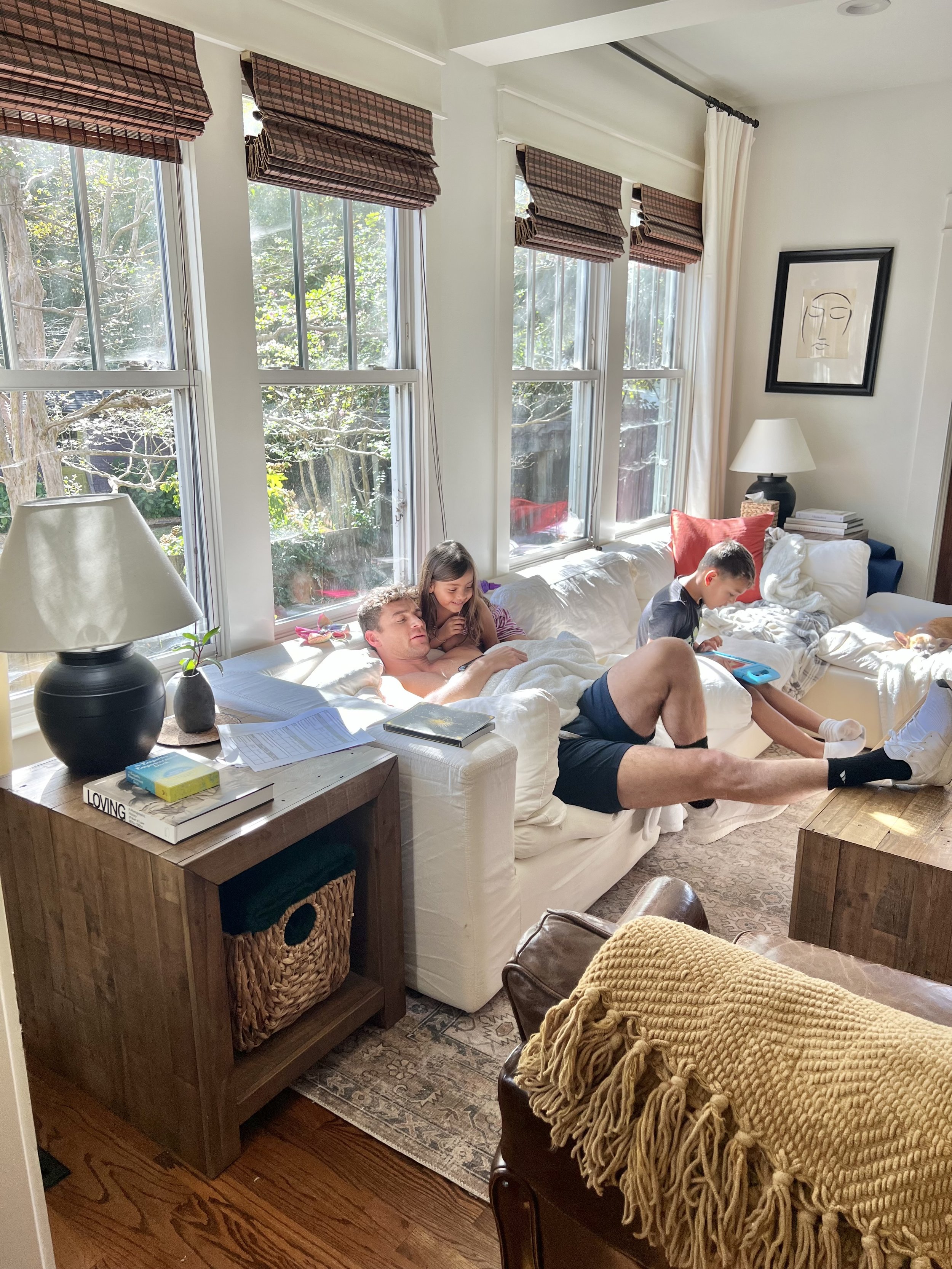In this bright and airy living room, sunlight streams through the four windows in the top left, illuminating the space and glinting off the blinds that are partially rolled up, revealing the green leaves of trees outside. Central to the scene is a pristine white couch where a man reclines with his feet propped up on a white wooden coffee table. He's dressed in shorts and socks, and beside him, a young girl is smiling and leaning against him, both engrossed in something he's holding, perhaps an iPad. To their right, a young boy is absorbed in playing with a blue device, likely a game on an iPad, with a red pillow just behind his head. Snuggled in the far corner of the couch, a tiny chihuahua naps in the sun. The couch is flanked by a wooden end table adorned with a black lamp and off-white lampshade. The floor is covered by a large, intricately designed grayish rug, with dark brown hardwood peeking around its edges. In the bottom right corner, a brown leather chair sports a tan blanket draped over its back, completing the comfortable and modern family room scene.